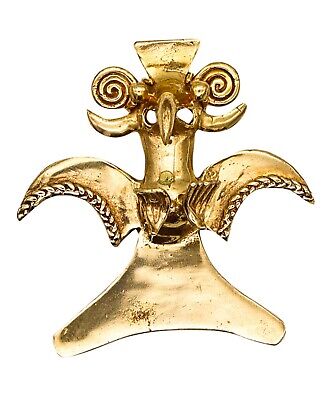The image depicts a small, antiqued gold artifact that resembles a bird or owl, possibly a pendant or statue, likely intended for use as a necklace or display item. The object’s upper part features a triangle that suggests it can be hung, paired with spirals that adorn the area beneath pointy ear-like projections. Prominently in the center, between two eye sockets, a beak extends forward. Below the spirals sit horn-like shapes, transitioning into a long, slender neck that culminates in feather-like or wing-like extensions. The body of the item has a detailed rope border design on winged appendages, resembling bird or bat wings. These wings jut out from the sides, adding to the intricate complexity of the piece. The base of the artifact is triangular and wishbone-shaped, resembling the claws or feet of a bird, providing stability if placed on a flat surface. The design exudes an ancient, possibly museum-worthy feel, with its detailed craftsmanship and singular golden coloration standing out against a neutral background.